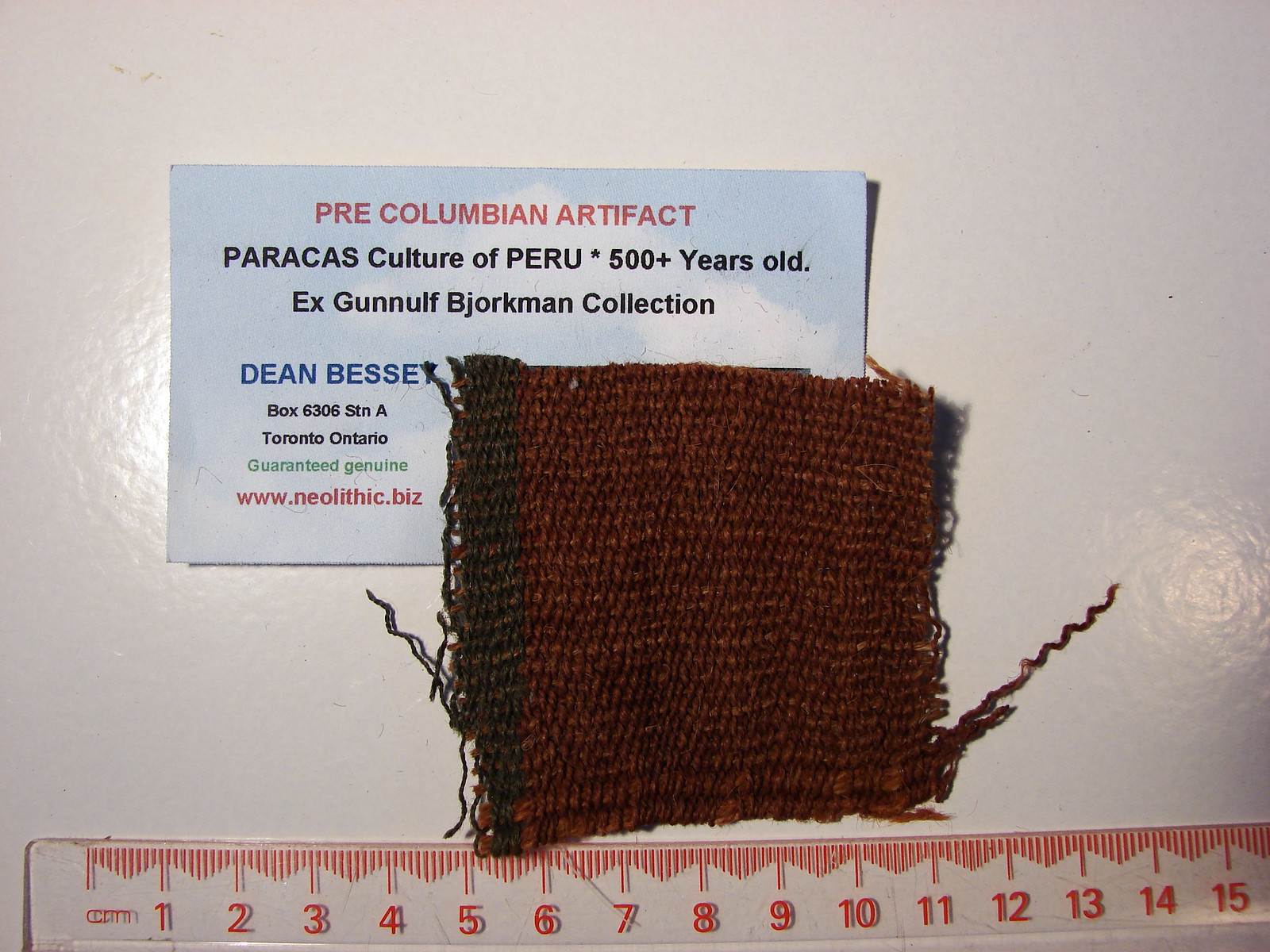The image depicts an aged and frayed square piece of brown fabric, positioned against an off-white background. Beneath this artifact, a transparent ruler featuring red lines and numbers measures its dimensions, highlighting that it spans from the 5 cm to the 11 cm mark. Behind the fabric, a white paper card is displayed, bearing red text at the top that reads "Pre-Columbian Artifact". Below that, in black text, it is labeled "Paracas Culture of Peru, 500 plus years old, Ex-Gunalof Bjorkman Collection." Further details on the card include a blue text identifying "Dean Bassett", with additional black text giving the address "Box 6306, SCNA, Toronto, Ontario." Green text assures "Guaranteed Genuine", and red text provides the website "www.Neolithic.biz".